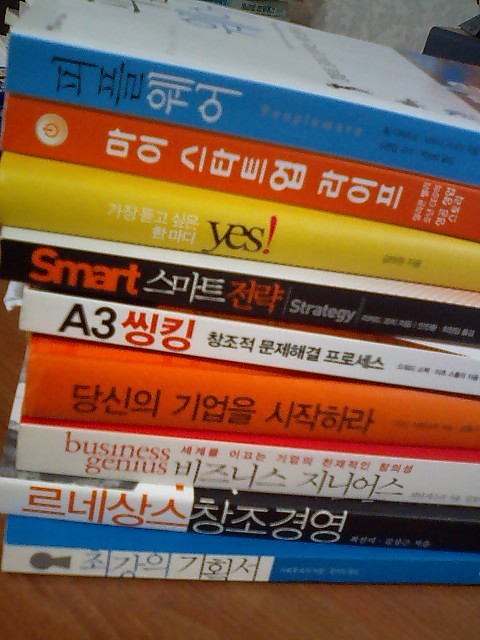The image features a neatly stacked pile of nine colorful textbooks, resting on a medium brown wooden surface, with a grey wall as the backdrop. The books are written in what appears to be Korean, although some details may suggest Japanese. Each book is about half an inch thick. Starting from the bottom of the stack, the books display a vibrant array of colors and English phrases amidst the non-English text. 

The bottom book has a blue spine, followed by a book with a predominantly white and black spine, featuring some writing in red and white. The next book has a white spine with "BUSINESS GENIUS" inscribed in red. Above it sits a book with a red spine, then one with a white spine that contains both black and red writing. Following this is a book with a black spine displaying the word "SMART" and "STRATEGY" in white letters, along with additional text in a non-English language. Next, there is a book with a yellow spine, prominently showcasing the word "YES!" in bold black letters. The stack continues with a book with an orange spine, and finally tops off with a blue spined book. These vividly colored spines make the stack visually striking and engaging.